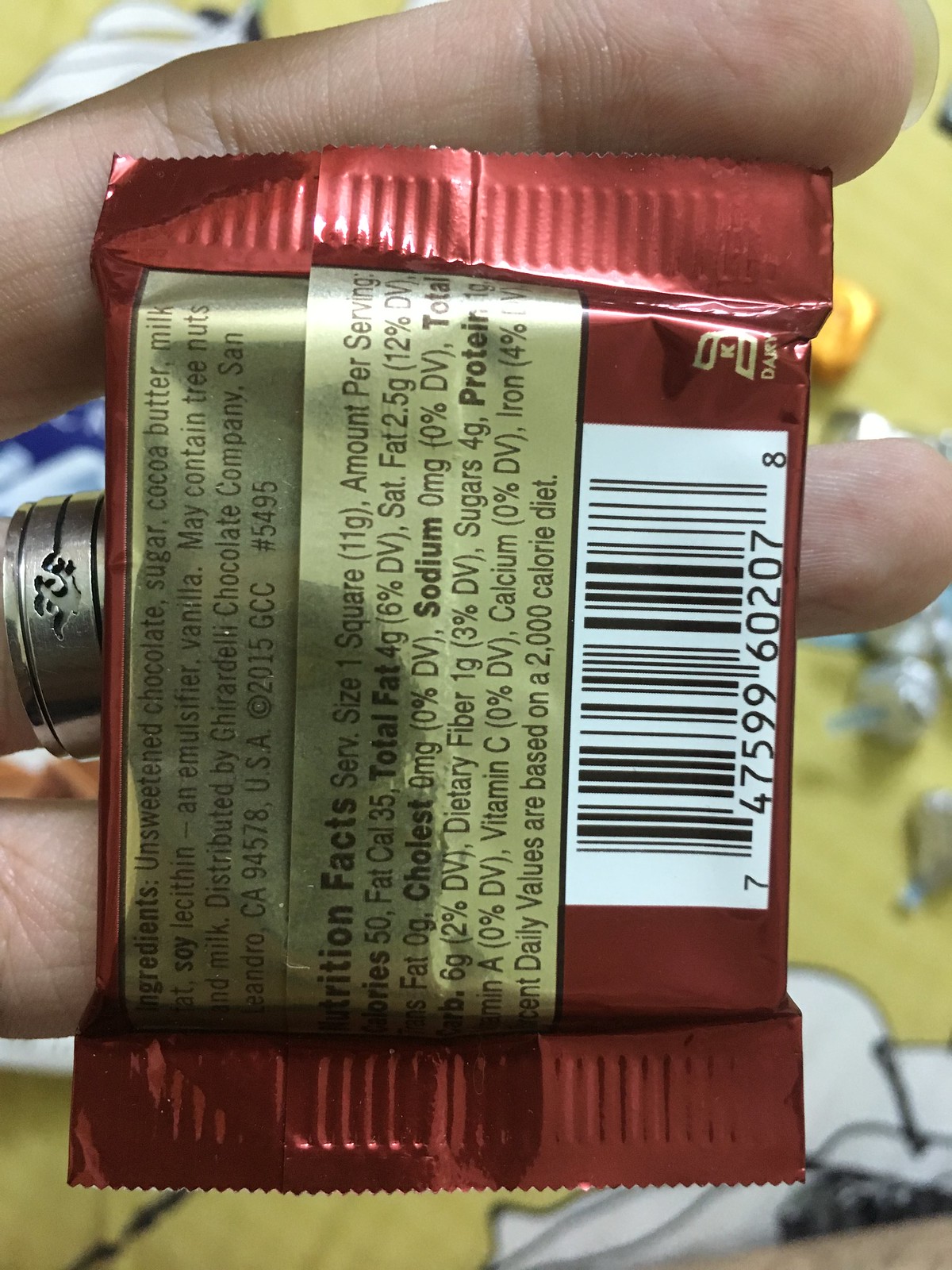In this image, a hand adorned with a detailed silver ring holds an individual piece of Ghirardelli chocolate at a slight sideways angle. The chocolate is wrapped in distinctive red packaging, with a barcode visible on the bottom. The opened wrapper partially covers the fingers of the hand. The label lists the ingredients: unsweetened chocolate, sugar, cocoa butter, milk fat, soy lecithin (an emulsifier), vanilla, and it notes that the product may contain tree nuts and milk. The chocolate is distributed by the Ghirardelli Chocolate Company, based in San Leandro, California. The bottom right-hand corner of the packaging features the word "dark," indicating that this is a square of Ghirardelli’s dark chocolate. This type of individual chocolate square is often found in bulk at retailers like Costco.